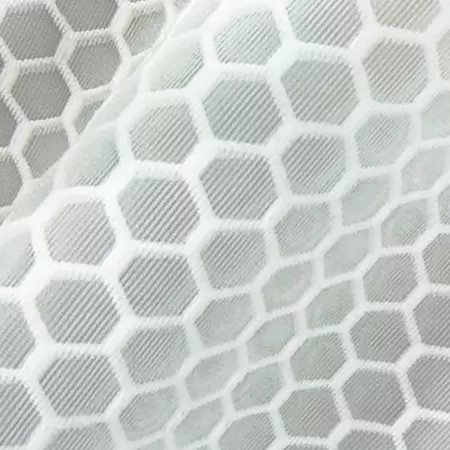The image depicts a detailed fabric pattern resembling a honeycomb structure, primarily composed of gray and white colors. The design features hexagonal shapes that look fuzzy, akin to pipe cleaners, and are arranged in a way that evokes the appearance of a honeycomb. The fabric appears to be billowing slightly, giving it a ruffled, non-flat texture, as if it's blowing or rippling in the middle. The interplay of light and shadow adds depth to the image, accentuating the pattern's dimensionality. The hexagonal shapes contain lines within each, contributing to the intricate design. The overall impression is of a complex, biologically-inspired textile with a dynamic, flowing quality.